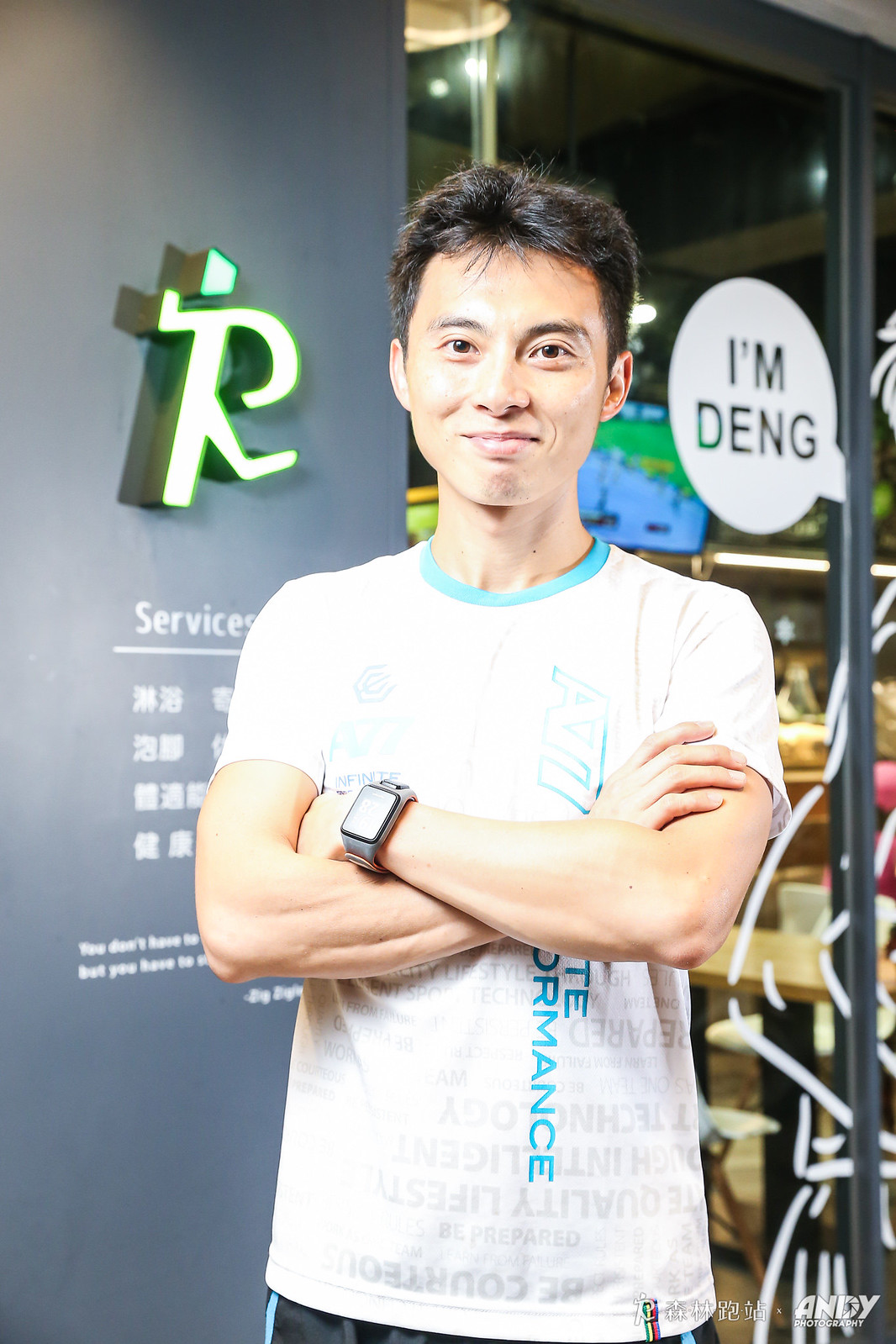This picture captures a young Asian man, approximately 30 to 35 years old, posing with a soft smile and his arms crossed. He has short black hair and is dressed in a white T-shirt featuring prominent blue text and trim at the collar, which also includes some faded grey text and a blue logo. A smartwatch adorns his left wrist, and he is wearing black shorts. Standing in front of a structure that appears to be a storefront, the background features a variety of distinctive details. Over his left shoulder, there is a grey wall displaying a lit-up, green running figure in the shape of the letter 'R', under which the word "services" is written alongside additional text in what appears to be Chinese or Japanese. To his right, a glass window displays a caricature with a speech bubble saying "I'm Deng" in black text. This image, potentially for a social media post, suggests that he may be part of a crew associated with the establishment.